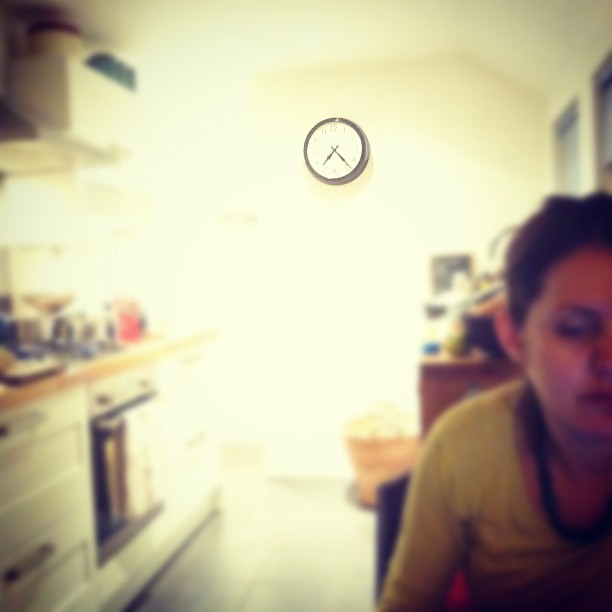In the image, a black-framed wall clock with a white face and black numerals is the primary focus. The clock, displaying 7:35, is positioned high on a kitchen wall. The photograph features a shallow depth of field, making the clock the only clear element, while the rest of the scene is artistically blurred. In the foreground, a little boy wearing a yellow shirt sits in the bottom right corner, his face illuminated with a blue tint, possibly from a tablet. To the left, a kitchen counter and shelves are visible, along with a built-in silver stove or oven and wood-grained drawers below. On the floor in the background is a large basket with two handles. A small picture adorns the wall to the right, and the white, angled ceiling leads to two tall, rectangular windows outlined in the top right corner of the image.